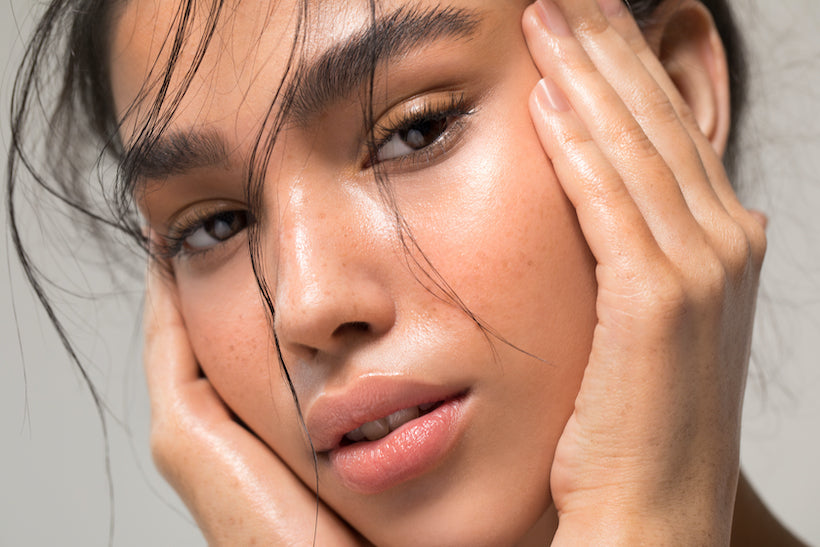The image showcases a close-up of a young woman’s face, framed from the neck upwards. Both of her hands are pressed against her cheeks, with her fingers extending out of the frame. Her head is slightly tilted to her right, giving a diagonal appearance, and she gazes towards the camera with the left side of her face more visible. She has dark, well-groomed eyebrows and thick, dark hair, which is mostly pulled away from her face, though a few strands cascade over her forehead and around her eyes. Her lips, lightly adorned with pink or coral lipstick, are parted to reveal her top front teeth. Her complexion has a light tan, and her hazel brown eyes reflect a soft glow from the lighting. The background of the image is a neutral, light gray, providing a subtle contrast to her lightly made-up visage.